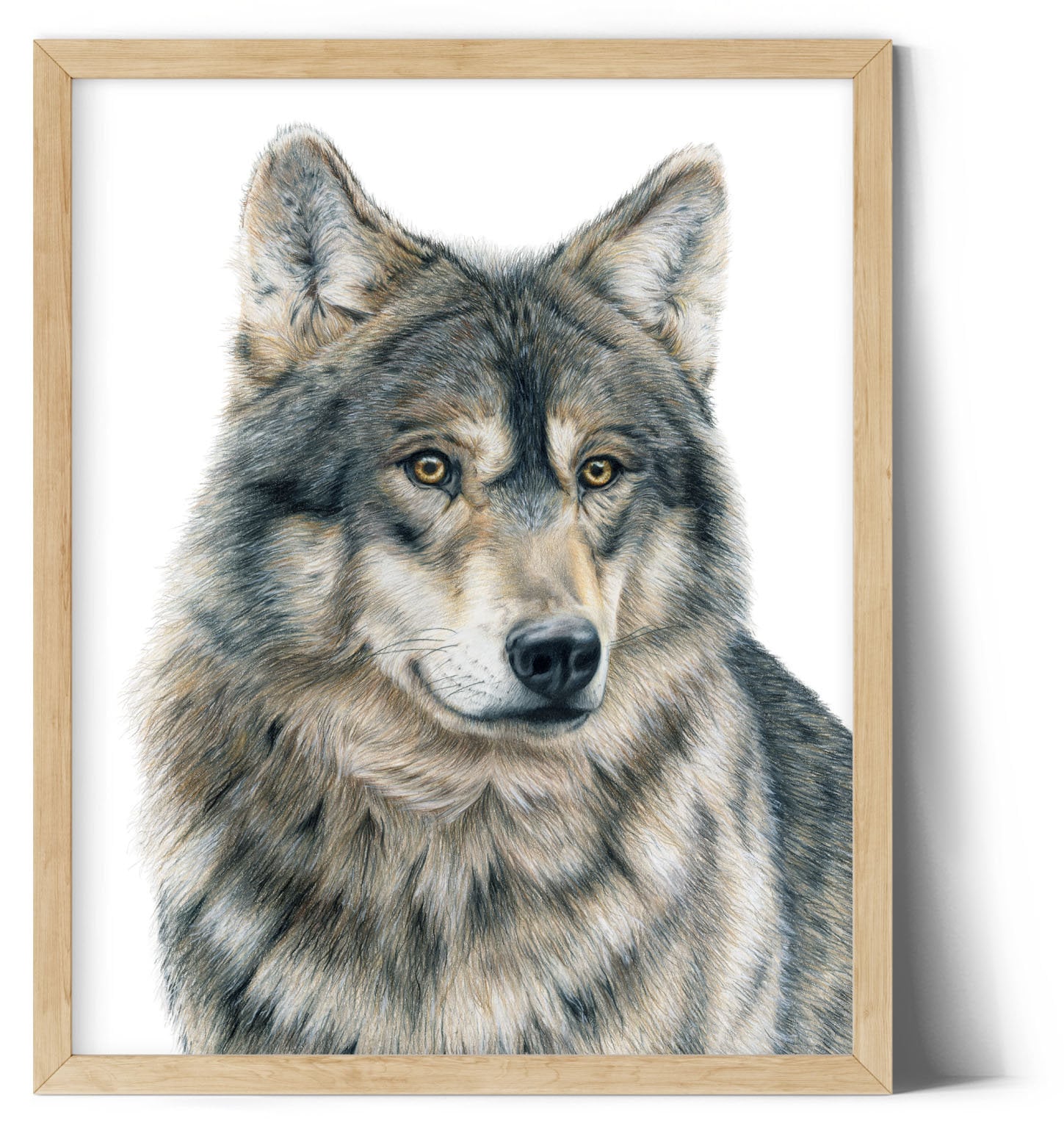This is a highly detailed painting of a wolf, meticulously rendered with attention to every strand of fur, giving it a bordering-on-photorealistic quality. Set against a plain white background, the wolf is the sole focus of the composition. The artist employed a range of colors including black, white, gray, and subtle touches of yellow, accentuating the wolf's realistic fur texture and the little brown nose. The eyes, though slightly off, add a unique character to the piece. Framed in an elegant wooden frame, the painting casts a discernible shadow on the wall behind, suggesting it was photographed from a ground-level angle, enhancing its lifelike appearance.